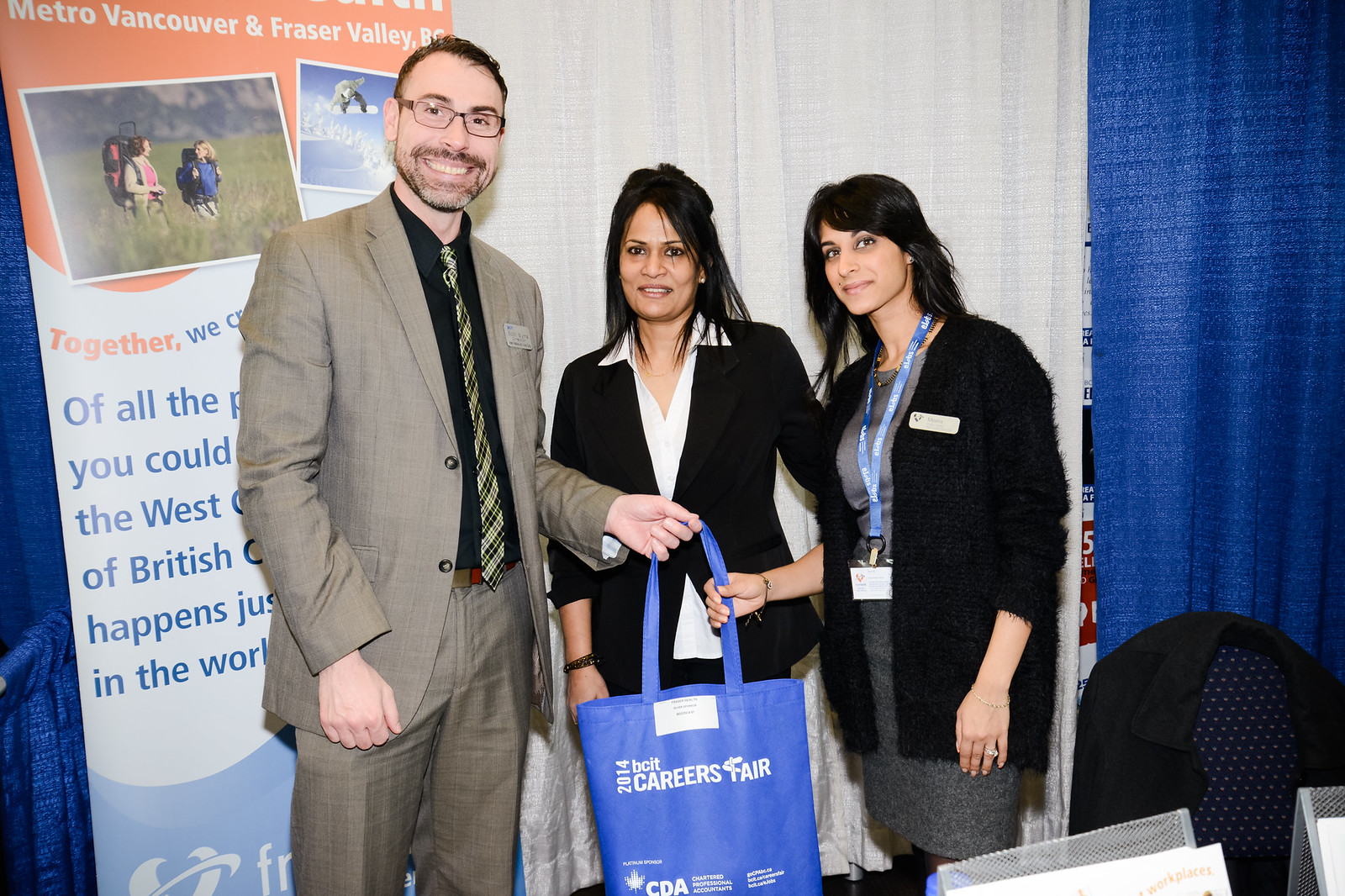In this image, three people stand posed in front of a white and blue curtain wall and a banner that highlights outdoor activities and reads "Metro Vancouver and Fraser Valley, BC" in white text at the top. On the far left is a tall man with brown-rimmed glasses, a short-cropped beard, and mustache. He is dressed in a tan-colored business suit, a black button-up shirt, and a yellow and black plaid tie. He is handing a blue canvas bag that says "2014 Boat Careers Fair" to a woman on the far right. The woman in the center wears a black coat over a white button-up shirt, while the woman on the far right is dressed in a black sweater jacket and a gray dress. The scene evokes a formal event, likely a careers fair, underscored by the professional attire and the informational banner in the background.